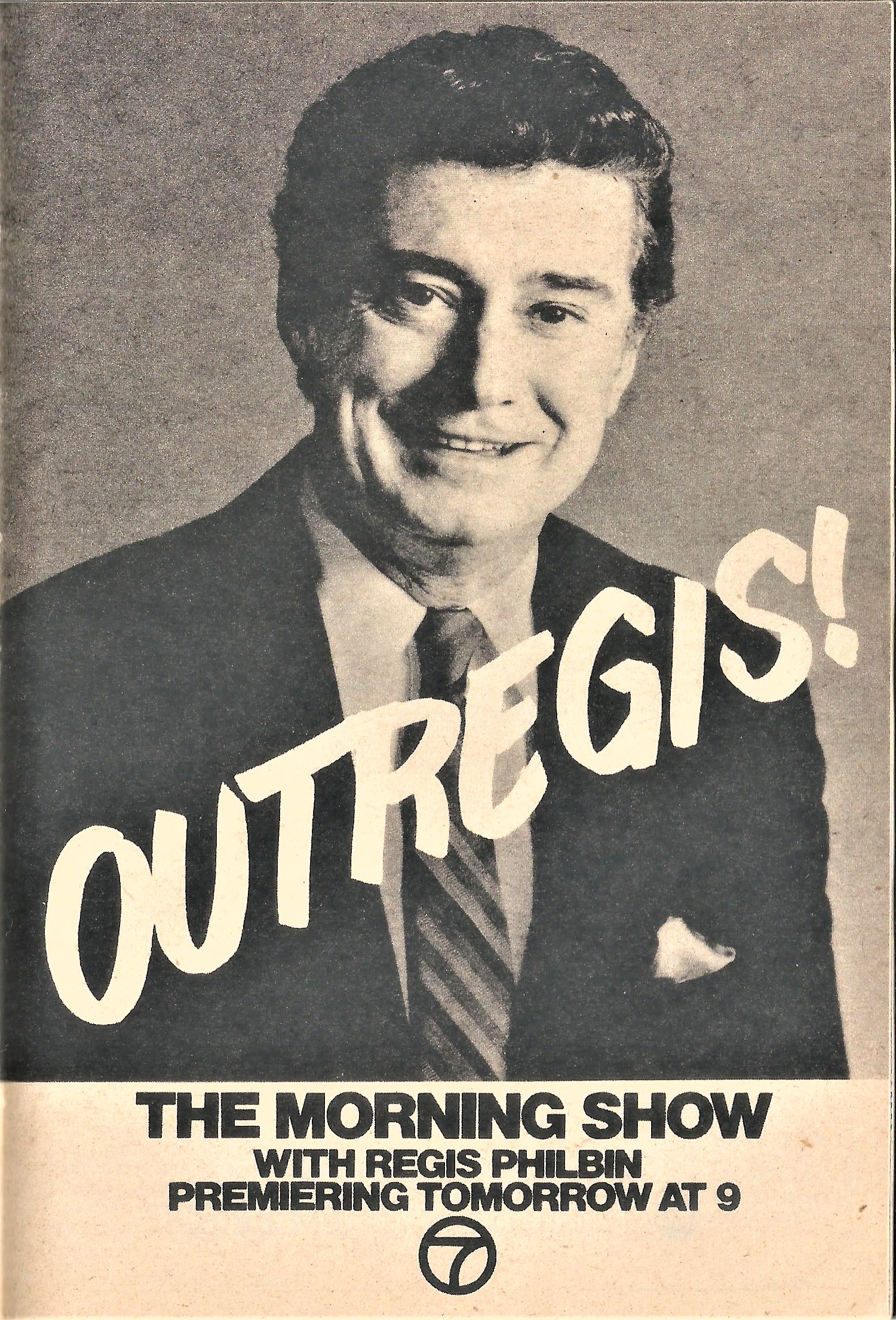This old-fashioned black and white advertisement features Regis Philbin prominently in the center against a light gray background. Regis is smiling at the camera, wearing a black suit jacket, a white shirt, and a multi-colored striped tie. A white pocket square adorns his breast pocket. His hair is dark and slicked back, and he is clean-shaven. Large white letters at an angle exclaim "Out Regis!" Below this, a white box with black letters announces "The Morning Show with Regis Philbin premiering tomorrow at 9." Additionally, a black circle with the number 7 is visible. The image resembles a scan of a magazine or newspaper page, providing a nostalgic look at the era.